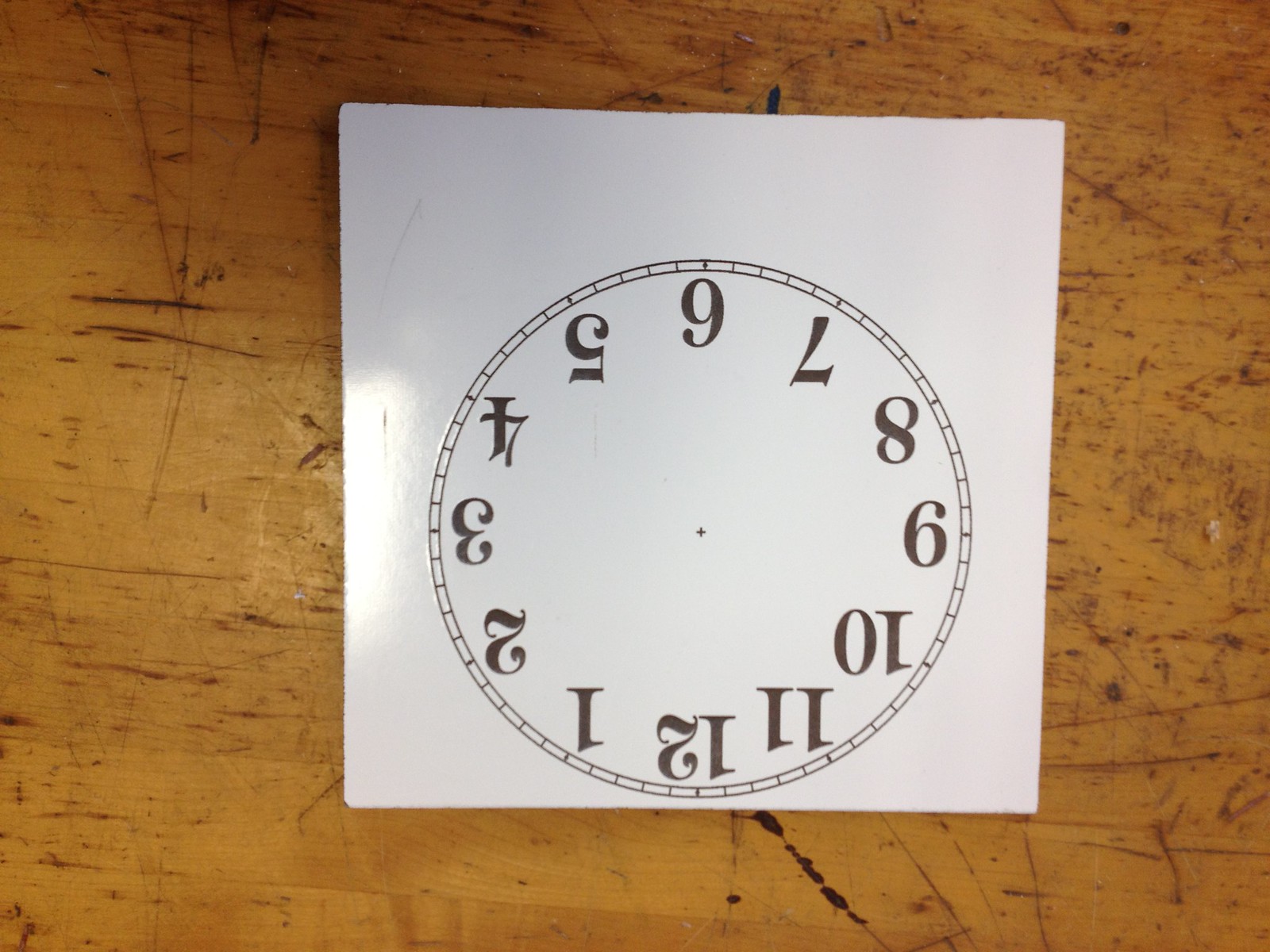The image depicts a square piece of white paper lying on a heavily scratched and distressed honey-colored wooden tabletop. The wood exhibits a blondish hue with dark brown distress marks and various scratches, suggesting the surface is old and well-used. On the paper, there is an outline of a clock face depicted in a serif font with numbers 1 through 12 arranged in a clockwise fashion. Notably, the clock face is upside down, with 12 o'clock at the bottom and 6 o'clock at the top. Surrounding the main circle of the clock is a smaller ring with minute markers, though no hands are present. A tiny cross or plus sign marks the center of the clock face. The overall scene gives the impression of a work-in-progress for a clock-making or teaching activity.